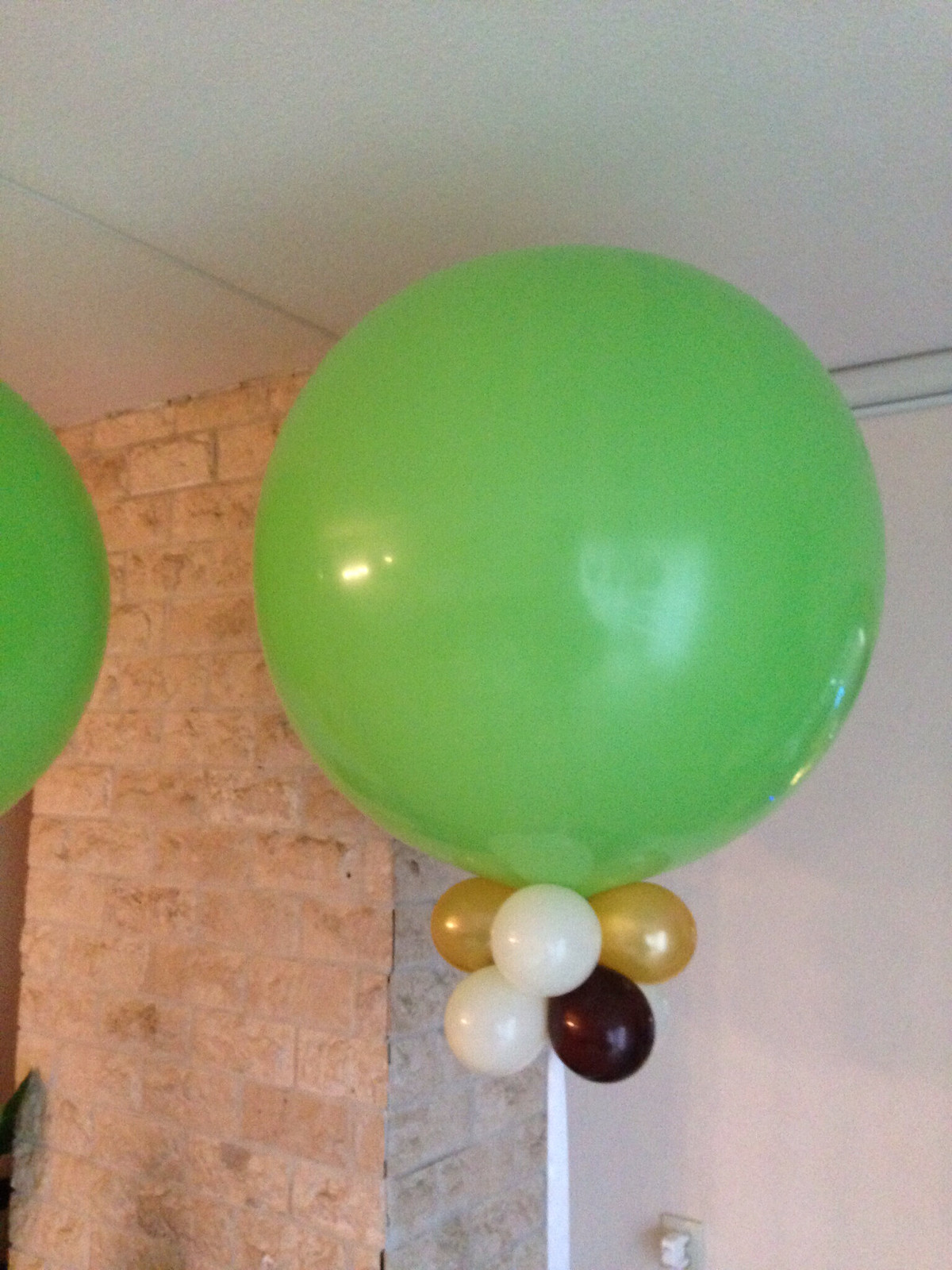This image is a photograph featuring a decorative arrangement of festive balloons. The focal point is a large, bright green spherical balloon positioned just right of center. Attached near the bottom of this main balloon is a cluster of smaller balloons in gold, white, and black hues. The background showcases a white wall on the right side of the image, while to the left, there is a large pillar made of lighter-colored brown brick. The white ceiling frames the scene from above. To the far left of the image, part of another similarly colored green balloon is visible, though most of it remains out of view, suggesting there might be multiple such arrangements, potentially assembled for a celebration. The overall composition and array of colors strongly hint at a festive and celebratory atmosphere.